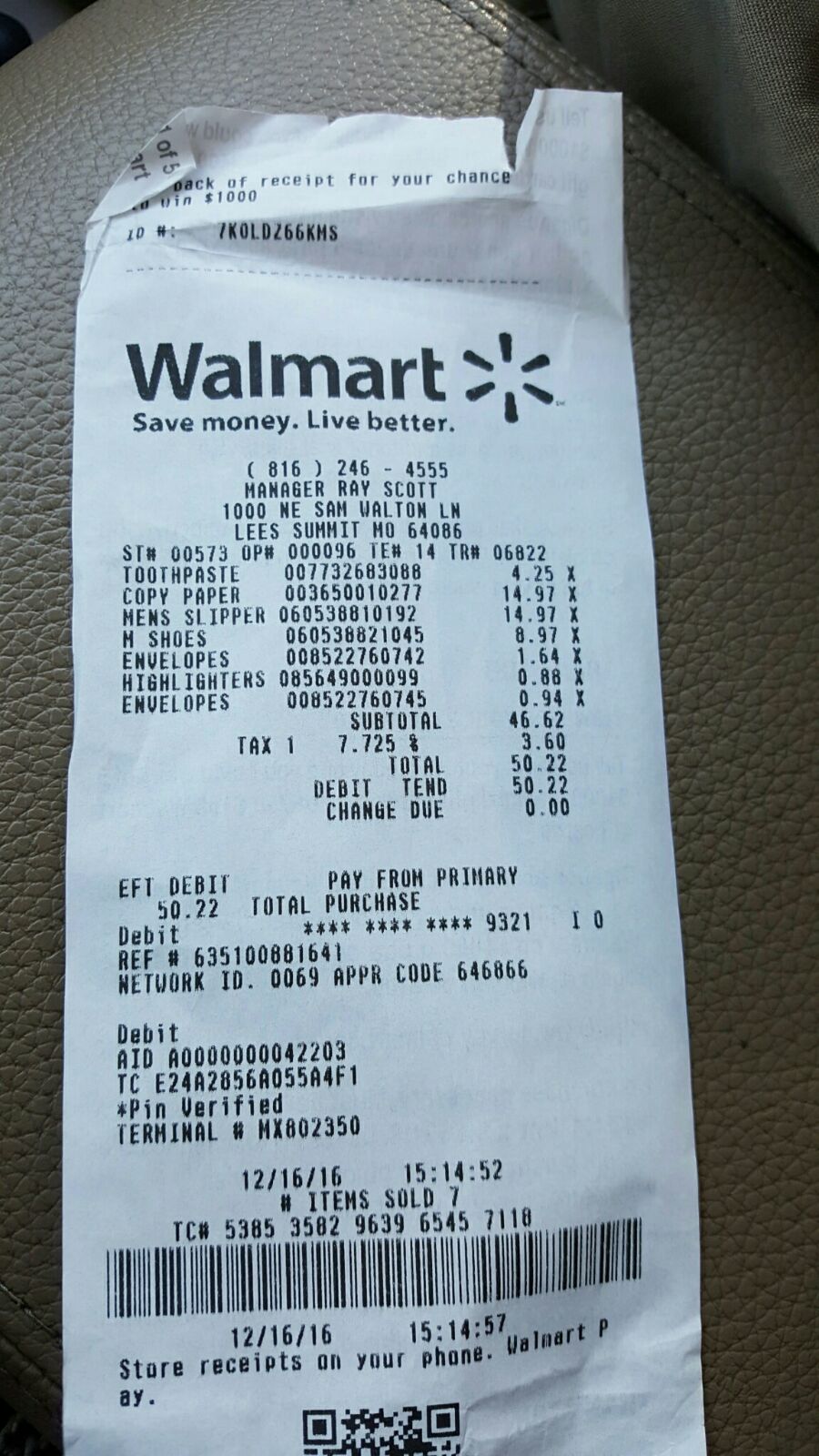A torn receipt sits on a medium-gray, reflective leather or pleather surface with black stitching, creating a textured backdrop. The top edge of the receipt is ragged, suggesting it was hastily torn. The receipt features the prominent "Walmart" logo in large black letters, accompanied by Walmart's distinctive circular icon to the right. The tagline "Save Money. Live Better." is printed just below the logo. Additionally, there is information about the store's location and contact details. The body of the receipt lists detailed information about the purchased items. At the very bottom, the date "12/16/16" along with the time "15:14:57" are clearly printed, marking the exact moment of the transaction.